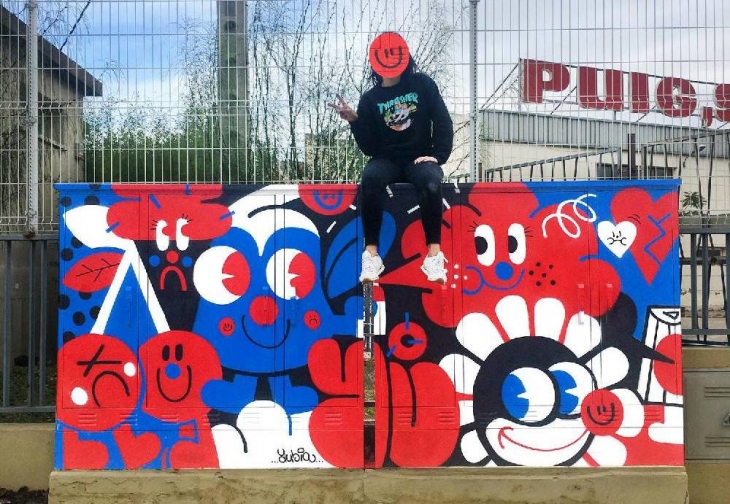This is a horizontally aligned rectangular photograph featuring a young woman sitting atop a sturdy, painted utility box adorned with vibrant cartoon patterns primarily in white, red, blue, and black. She is dressed in a black hoodie with a graphic image and the word "Thresher" on it, black leggings, and white tennis shoes. The woman’s long black hair is visible, though her face is obscured by a red circle with a hand-drawn smiley face. Her left hand rests on her thigh while her right hand is extended doing a peace sign. The cartoon designs on the utility box include a large, animated creature with short legs, big eyes, and a big smile, along with oversized flowers and a sun. The scene is set against a tall wire fence, with industrial buildings in the background. One building prominently displays a partially visible sign that reads "PUIG."